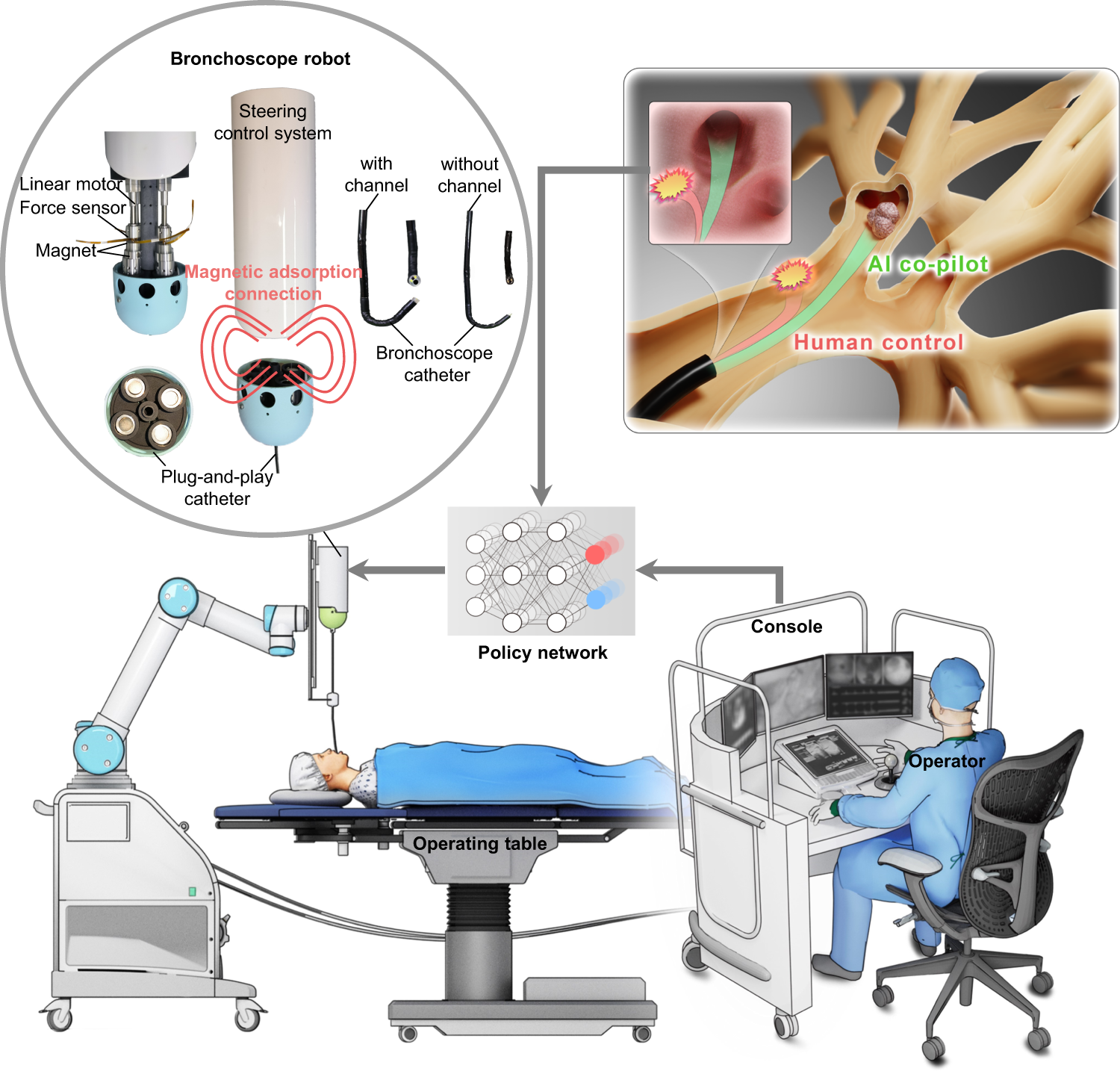This detailed color diagram illustrates a robotic surgical system focused on a Bronchoscope robot used in lung procedures. In the top left, there's a circular inset showcasing close-up details of the Bronchoscope robot's components, including a linear motor force sensor, a magnet, a plug-and-play catheter, and a magnetic absorption connection, alongside Bronchoscope catheters with and without channels. Adjacent to this is a rectangular inset depicting a scanner entering light brown lung tissue, highlighting the branch-like texture of the lungs. This section is annotated with "AI copilot" in green and "Human control" in red. Below these insets is the main image: a patient in a blue hospital gown and cap lies on an operating table, covered with a blanket, with a large robotic machine's arm extending a tube into their mouth. This central part of the diagram illustrates a complex "policy network" with numerous interconnected nodes. Beside the patient, a doctor in scrubs is seated at a rolling desk in an office chair, operating a console with three computer screens, engaged in controlling the surgical procedure.